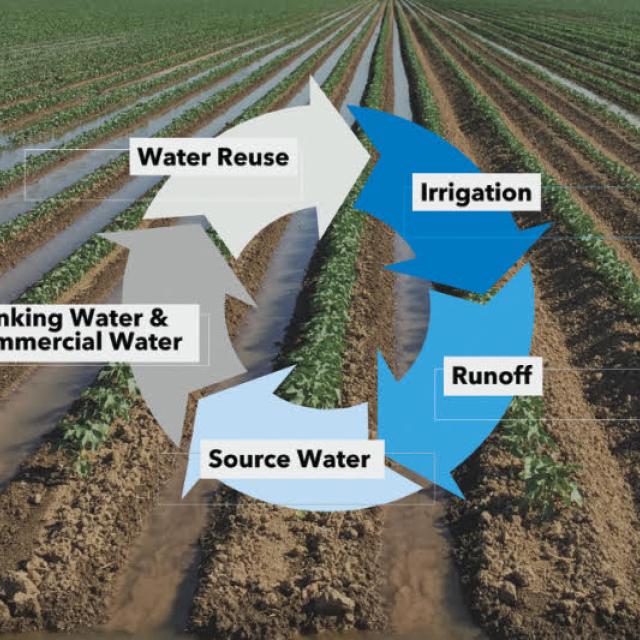The image depicts a detailed agricultural scene featuring rows of crops growing in a furrowed field, with water visible between the mounds of soil. Superimposed on this photo is a cyclical diagram that illustrates the process of water reuse in agriculture. Despite its pixelated quality and some text being partially cut off, the diagram uses various colored arrows to indicate different stages in the water cycle. The blue arrow labeled 'irrigation' points to a lighter blue arrow marked 'runoff,' which then leads to another lighter blue arrow indicating 'source water.' This water transitions into 'drinking water' and 'commercial water,' represented by a gray arrow, though part of this text is obscured. A white arrow labeled 'water reused' completes the cycle by directing back to 'irrigation.' This visualization effectively illustrates the continuous loop of water use and reuse in the agricultural sector.